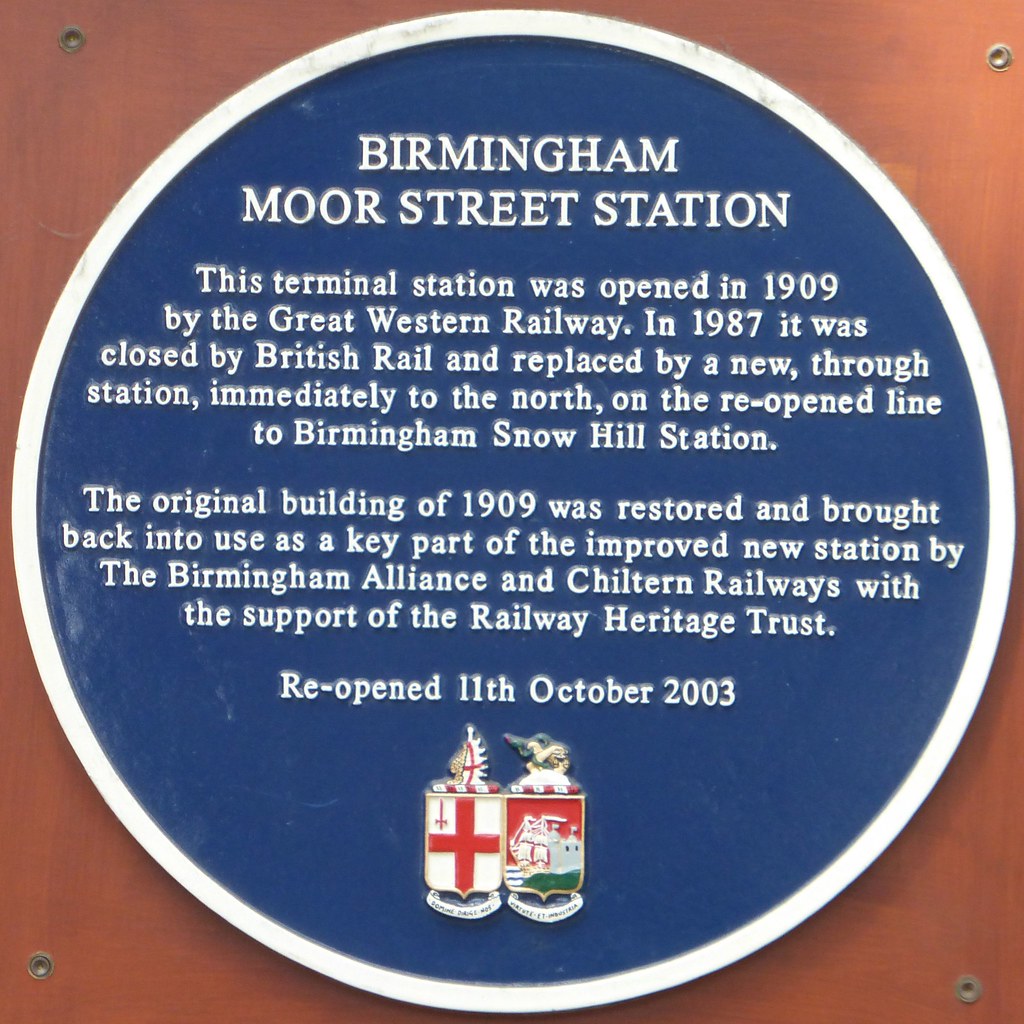This photograph features an informational plaque with a rusty, reddish-brown metal background, complete with rounded corners and screw holes. At the center of the plaque is a large circular emblem, consisting of a black, blue, and white border that nearly touches the edges. Inside the circle, white text reads: "Birmingham Moor Street Station."

The text provides a brief history of the station, stating: "This terminal station was opened in 1909 by the Great Western Railway. In 1987, it was closed by British Rail and replaced by a new through station immediately to the north on the reopened line to Birmingham Snow Hill Station. The original building of 1909 was restored and brought back into use as a key part of the improved new station by the Birmingham Alliance and Chiltern Railways with the support of the Railway Heritage Trust. Reopened 11th October 2003."

Beneath this, there are two coats of arms: one featuring a cross and the other a ship. Both crests are detailed with additional elements; one depicts arms, while the other shows a banner with the letter 'A.' The orange-hued backdrop adds to the plaque's vintage aesthetic.